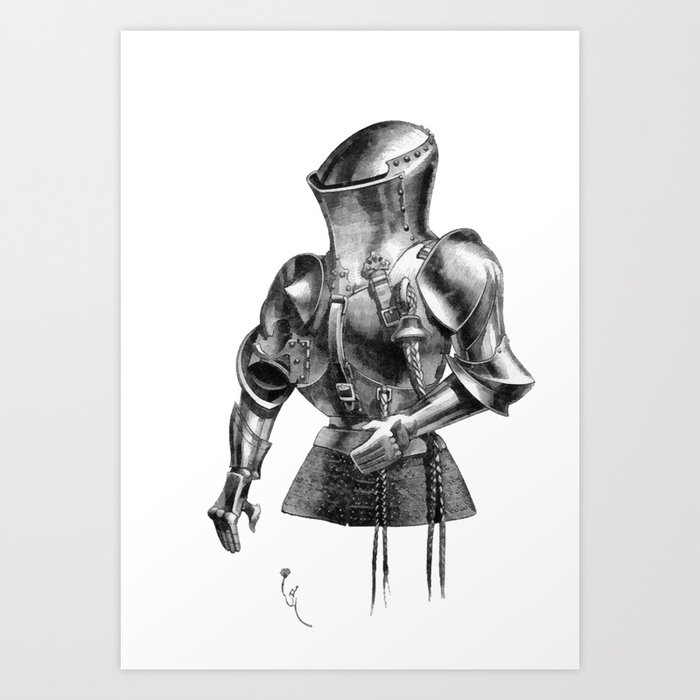This artist's depiction of a knight's armor captures a detailed and elaborate design. The drawing, presumably rendered in charcoal or pen and ink, sits against a white background, and showcases an intricately drawn medieval combat attire with a potential futuristic twist. The upper half of the armor covers the chest, back, neck up to the chin, arms, and includes hand areas designed for protective gloves. Detailed in silvery-gray, charcoal gray, and black, the armor demonstrates meticulous attention to light and shadow. Notably absent is the helmet that would complete the piece. The left hand is depicted bent at nearly a 90-degree angle with an open palm, while the right arm hangs relaxed at the side with fingers folded slightly and the thumb at a 90-degree angle. Decorative elements include two braids hanging from the belt on the left side, each braid splitting into two additional braids terminating in tassels. Additionally, a knife holder is visible on the chest, and two small, indeterminate silver squiggly lines are located below the armor to the viewer's left. The overall craftsmanship suggests a blend of historical medieval and speculative futuristic influences.